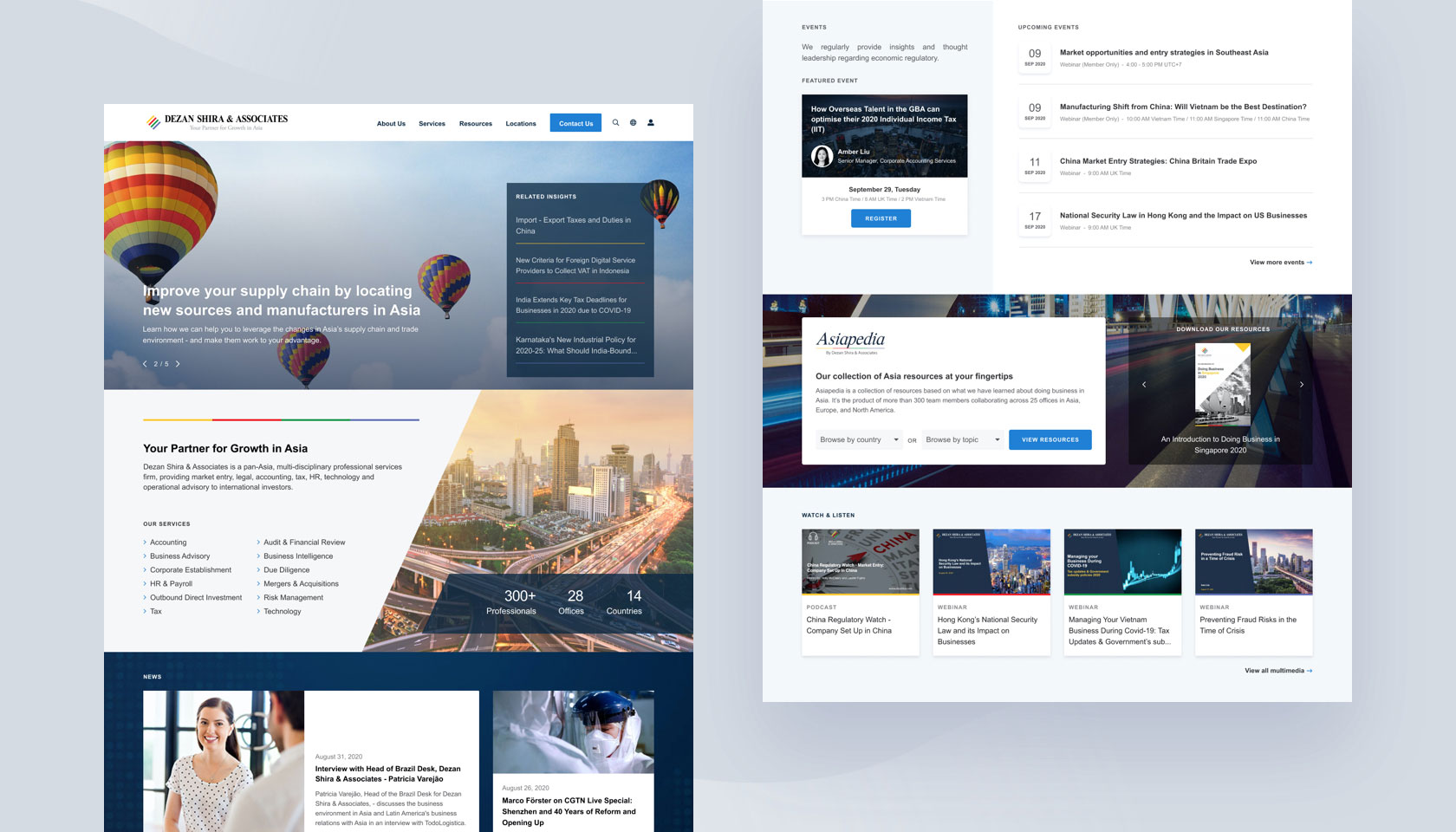The image showcases two website pages displayed on a rectangular backdrop, characterized by a black to medium gray gradient. The rectangle is horizontally elongated, with two distinct sections: one on the left and one on the right.

On the left side, the page prominently features the title "Dezan Shira & Associates" in large, bold black font. Below this title, there is some additional text in a very small gray font, which is difficult to read due to its minuscule size.

To the right, the webpage includes several navigational headings such as "About Us," "Services," "Resources," and "Locations." There is also a blue "Contact" button alongside a search icon shaped like a magnifying glass, a Facebook icon, and what appears to be a profile icon. This section is set against a white background.

Beneath the navigation links, a vibrant photograph depicts four hot air balloons drifting through a partly cloudy blue sky. The image caption, written in the largest font, states, "Improve your supply chain by locating new sources and manufacturers in Asia." Below this, a subtext in smaller font reads, "Learn how we can help you leverage the changes in Asia's supply chain and trade environment to work in your favor."

The right page has a taller than wide teal rectangle featuring white font. The precise content of this teal section is not specified.